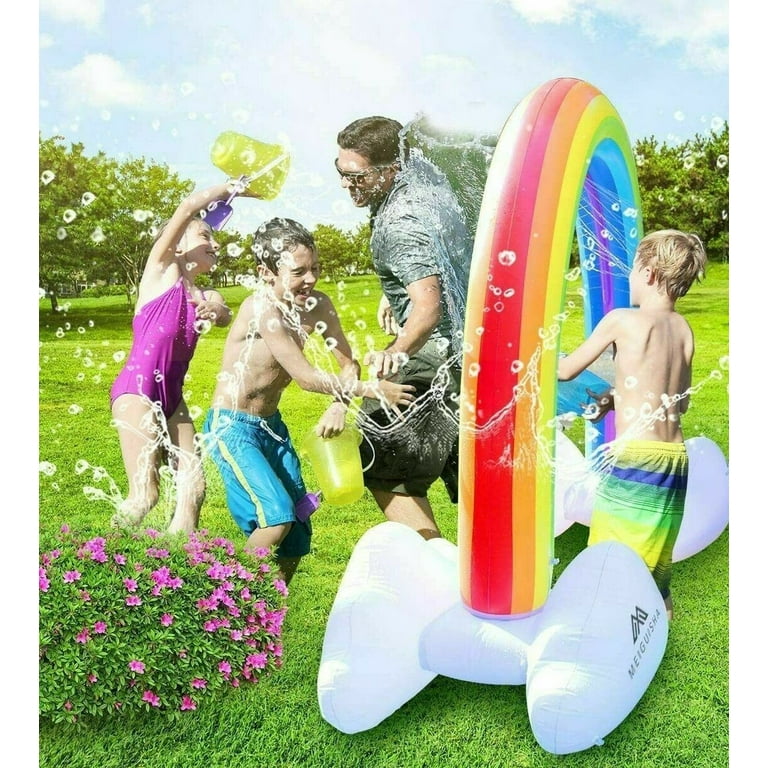In this vibrant and playful scene, we see a photo capturing a joyous outdoor moment on a beautiful day with a clear blue sky. Four individuals - an adult man in a gray T-shirt and shorts, and three children in colorful swimwear - are delighting in the spray of a tall inflatable rainbow sprinkler. The rainbow arches high with streams of water cascading from its top, anchored by white, cloud-shaped bases. One girl, dressed in a purple bathing suit, is poised to douse a boy in blue swim trunks with a yellow pail of water. Another child, the smallest boy, runs gleefully through the arch of the rainbow, while the third child heads towards the sprinkler, adding to the lively chaos. They are all situated on an artificial-looking green grass lawn, surrounded by flowering trees and a plant with pink flowers, giving the scene a manufactured yet picturesque park-like atmosphere. The playful setting is emphasized by the colorful inflatable, which could be a product photo for the sprinkler, bearing a partially visible logo that starts with an 'M'. The father, seemingly both partaking in and managing the fun, adds to the feel of family togetherness in the midst of water and bubbles flying everywhere.